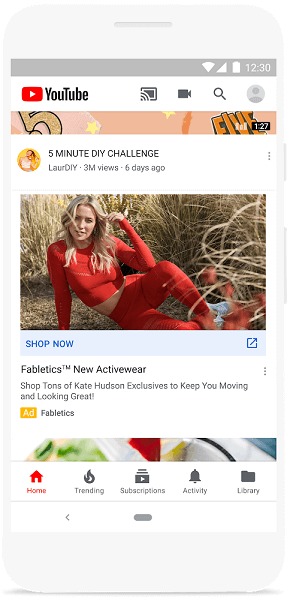A detailed caption for the described image could be:

"This image showcases a smartphone, predominantly in a whitish-gray color, with a visible power button and volume rocker located on its right side. Both buttons are light gray in color. The phone casts a shadow at its bottom, adding depth to the image. The screen displays a screenshot of the YouTube home screen. At the very top of the screen, within a gray rectangular strip, various icons indicate full Wi-Fi strength, a complete data bar, and a full battery, along with the current time, showing '12:30' in white text. Next to these icons, the YouTube logo is prominently displayed in black text, accompanied by a cast icon, a camera icon, and a magnifying glass icon, all in gray. The default gray profile icon denotes that no profile has been set. Below this, a series of thumbnails are visible, including an image of a girl in a red top and red pants with white shoes and blonde hair. An icon labeled 'SHOP NOW' in blue text and a blue launch icon are positioned at the bottom right of this image."